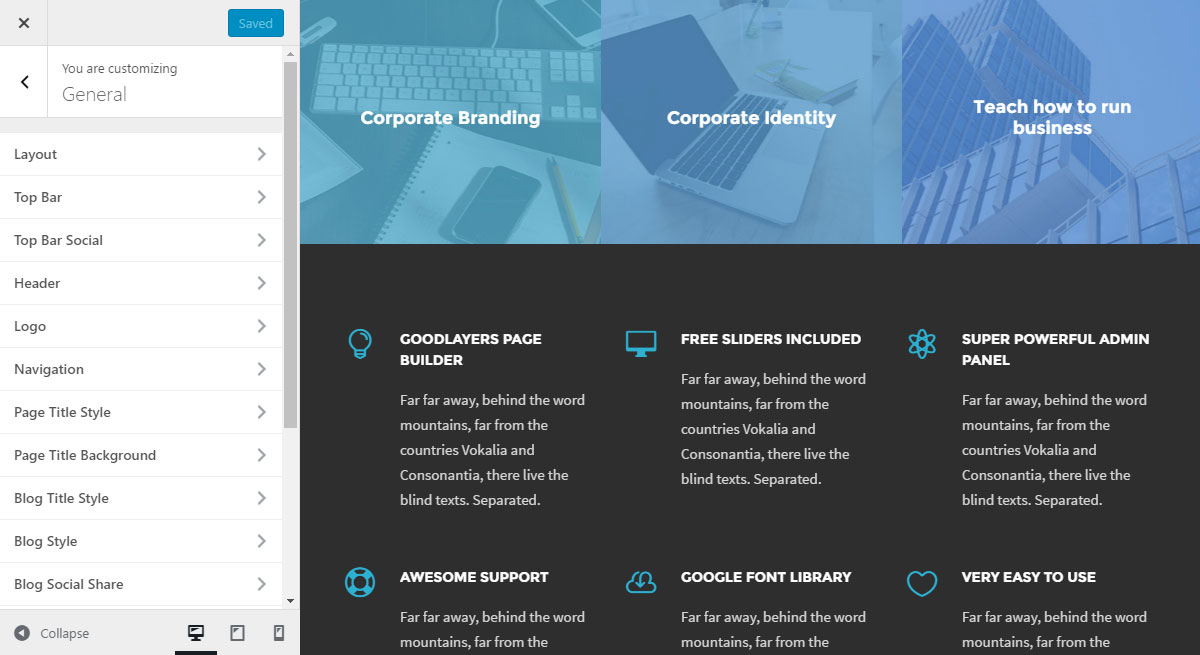The image displays a user interface for a customization tool. On the left side, there is a small gray box with a black "X" at the top, followed by a small blue box labeled "Saved." Below that, a small white box shows a left-facing arrow next to the text "You are customizing: General." A large gray line separates these elements from the rest of the interface. To the right of this line, there is a gray scroll bar and a vertical list of sections, each separated by thin gray lines and ending with right-pointing arrows. The sections include: Layout, Top Bar, Top Bar Social, Head Bar, Header, Logo, Navigation, Page Title Style, Page Title Background, Blog Title Style, Blog Style, and Blog Social Share.

At the bottom left, there is a small gray box with a circular icon and arrow labeled "Collapse." Underneath a black line, the content continues with visual elements: a computer screen, a page, and a phone icon. On the right side of the interface, a large box is divided into a blue top section and a black bottom section. In the blue section, various images of computers and buildings are accompanied by white text that reads "Corporate Branding, Corporate Identity," and "Teach How to Run Business." The black section includes a blue light bulb icon and white text that states "Good Layers Page Builder" next to a paragraph of text.

Adjacent to this, a computer screen graphic exhibits a blue and white color scheme with the text "Slide Free Sliders Included" in white. Another icon resembling an atom is labeled "Super Powerful Admin Panel" in white. Lastly, a tape graphic reads "Awesome Support" in white, next to text that mentions "Google Font Library" and an icon of two people in blue, alongside a blue heart icon and the phrase "Very Easy to Use."